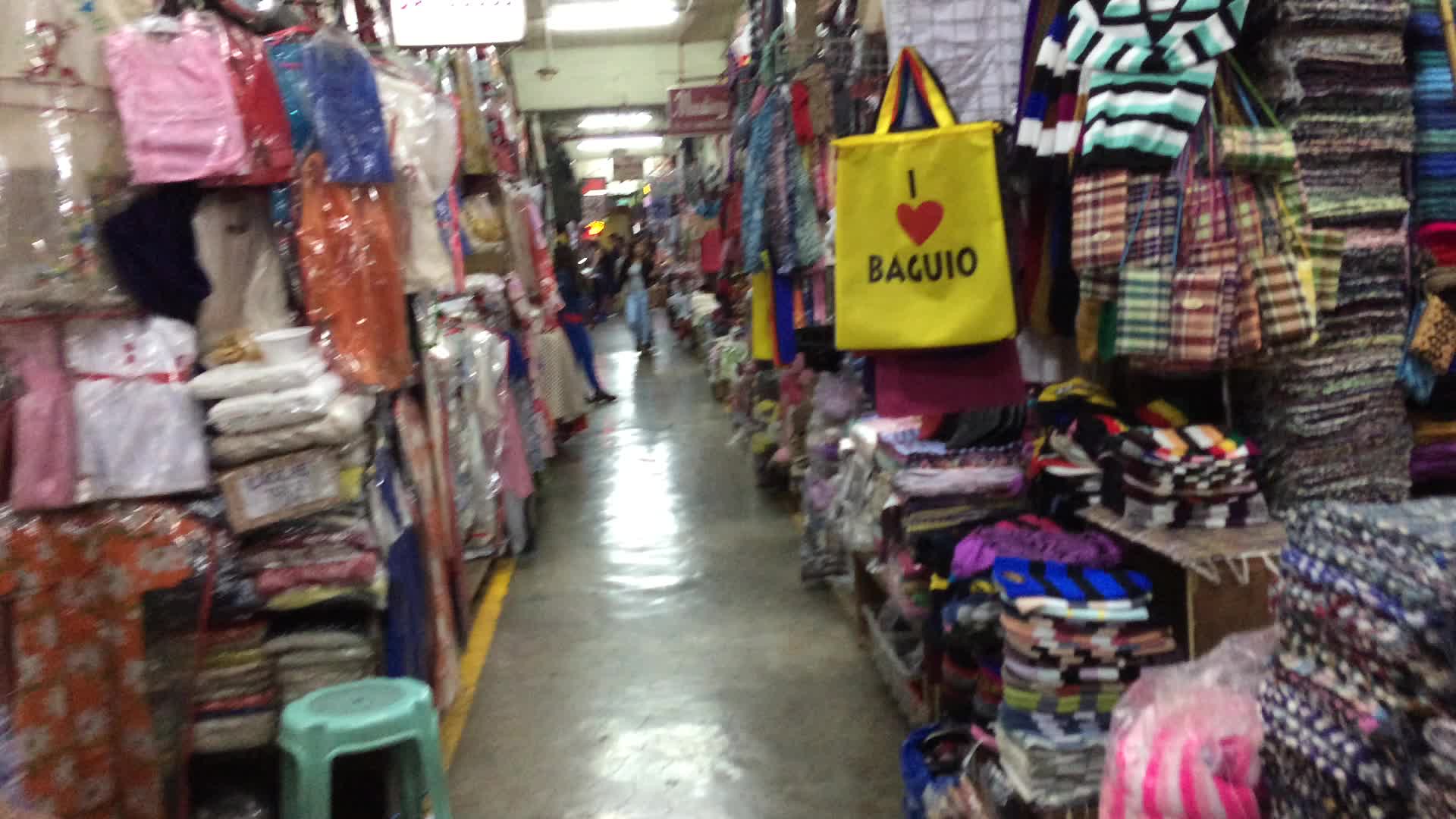This detailed image depicts an indoor marketplace with a shiny, hard concrete walkway positioned centrally. Various products, predominantly clothing, are meticulously arranged on shelves and hanging from hooks on both sides of the walkway. The vibrant display includes items in yellow, black, red, pink, orange, blue, light blue, tan, gray, and dark blue. On the left side, a little green step stool is visible beside shelves of folded and bagged materials, including some hanging white dresses. The right side mirrors this abundance with more stacked and hung garments. In the background, several people can be seen walking through the marketplace. Although most text is indistinguishable, a readable part on one of the bags says "I heart Baguio." The entire scene is illuminated by overhead lights, emphasizing the colorful assortment of goods in this bustling indoor shopping area.